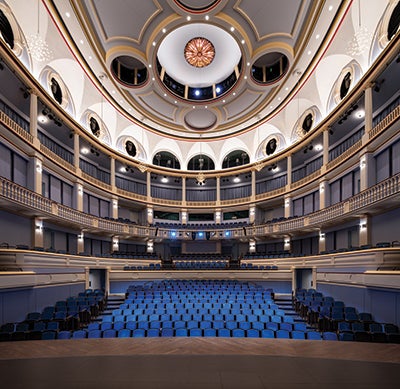The image captures an opulent, grand theater from the stage perspective, showcasing an empty auditorium with its rich architectural details. The seating arrangement is divided into three main sections of blue fabric chairs on the ground level, complemented by additional rows of seats on the balconies that span up to four levels. The theater's design is a semicircle pattern featuring ornate elements in stone, white, and gold, with large pillars encircling the space. The ceiling is domed and decorated with intricate gold accents, housing a prominent circular window, four smaller circular windows, and a grand chandelier. The scene suggests it is nighttime, as the windows reveal a black backdrop. The ambiance is subtly illuminated by three blue lights positioned at the back center of the theater.